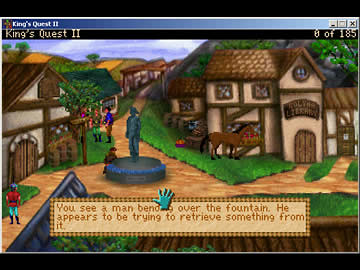This is a detailed screenshot of the classic point-and-click adventure game King's Quest 2. The game's title is prominently displayed in white text on a blue window bar at the top of the screen. The scene depicts an old-style town with beige buildings, wooden doors and windows, and light brown roofs. Surrounding the buildings is a grassy area interspersed with a tan-colored walking path that leads into a central courtyard. Dominating the courtyard is a gray statue of a figure. A text box at the bottom narrates, "You see a man bend over the fountain; he appears to be trying to retrieve something from it." A blue hand cursor hovers above this text box.

On the middle left, there is a statue of a bending figure, which the text describes, while the right side features a two-story house with a horse gazing inside. The intricate details include a series of mountains in the background and a walkway under an overhang or tent-like structure. The top right corner of the screen indicates "0 of 185," suggesting the start of an adventure. The immersive environment captures the essence of the game's intricate storytelling and atmosphere.